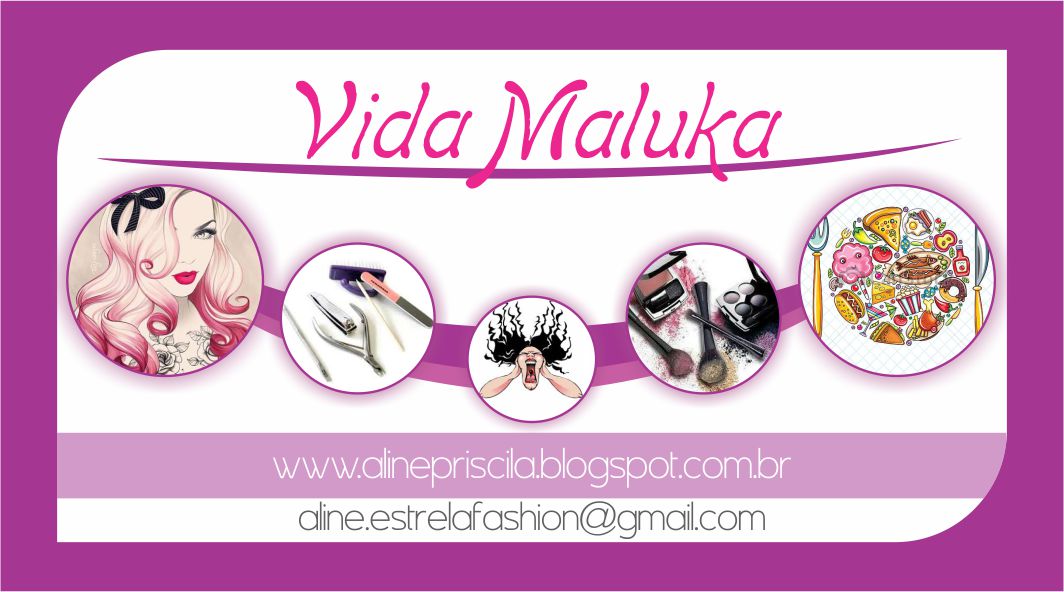A vibrant rectangular banner for a store, with a purple-violet border, showcases the brand name "Vida Maluca" in pink font on a curved purple line at the top. Below the title are five circular images: the first circle features a woman with long wavy hair, a black butterfly tie, bright red lipstick, and a floral patterned top; the second displays a set of nail clippers and nail care tools; the third, an animated woman with very long curly hair flying backward, screaming with her mouth wide open; the fourth circle contains an array of cosmetic powders and makeup tools; and the fifth depicts a plate loaded with various colorful foods including pizza and a donut. Beneath these images, the website www.alan9priscilla.blogspot.com.br and the email alan9astrofashion@gmail.com are displayed in black text.